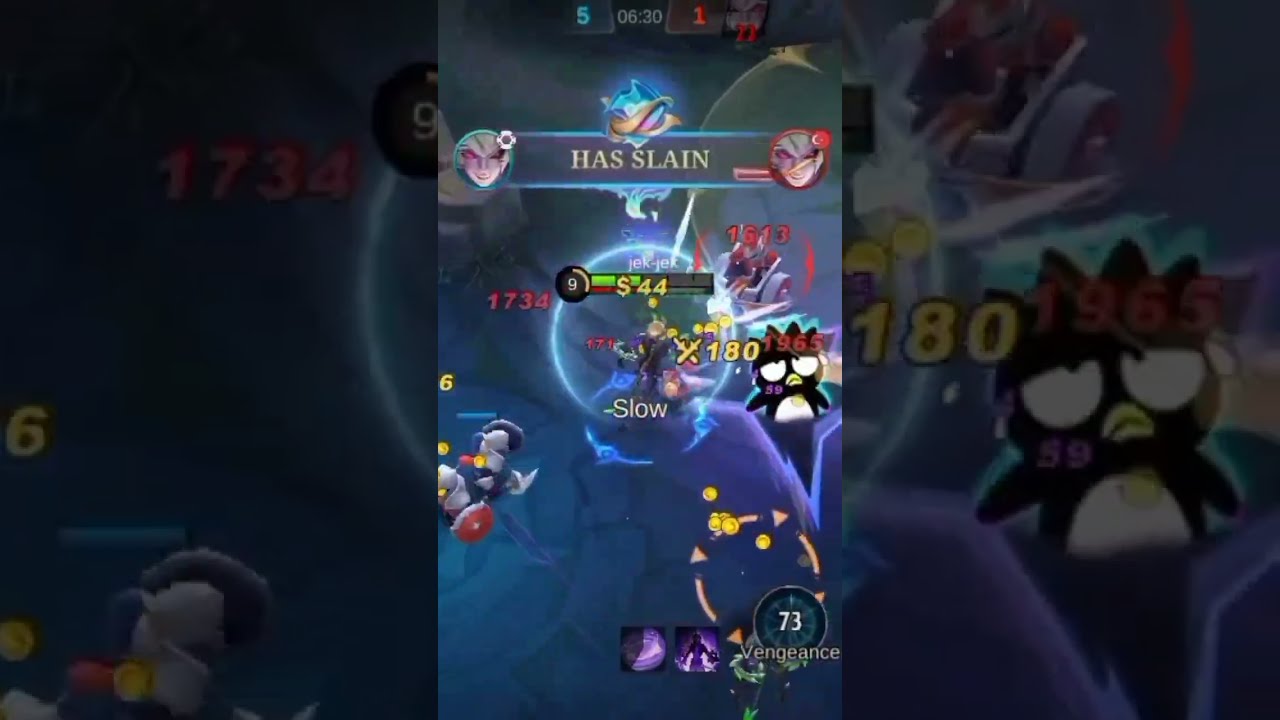This is a vertical screenshot of a mobile game that closely resembles League of Legends, possibly a spin-off or inspired version. The image features a blue and dark blue color scheme with an intricate User Interface (UI) optimized for mobile play. At the top center of the screen, an announcement reads "has slain," flanked by character icons. The middle section shows a bubble with the word "slow" and various combat-related numbers and debuffs, indicating real-time action such as damage dealt and received, and rewards earned. Lower down, iconic characters like Donald Duck and Hello Kitty’s Batsmaru appear, possibly as thematic in-game elements or overlays. The bottom right corner of the UI displays a mini-map and another circular icon with the number "73" and the word "vengeance." Enlarged, darkened versions of the Donald Duck and Batsmaru characters are used as side images on the left and right margins of the screenshot.